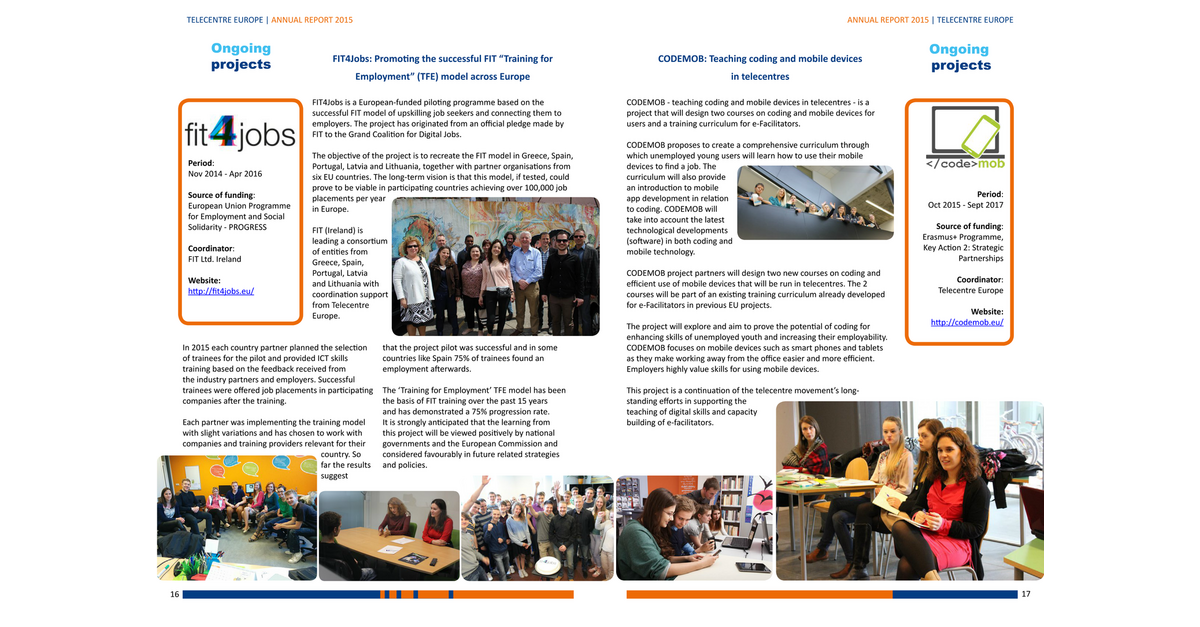The image is a screenshot of a website or a digital page from the Telecentre Europe Annual Report 2015, focusing on ongoing projects with a plain white background. The upper left side has "Telecentre Europe" in black and "Annual Report 2015" in orange, while the phrase "Ongoing Projects" appears in blue below it. Featured prominently is the "Fit for Jobs" project, promoting the successful Fit Training for Employment (TFE) model across Europe, detailing a period from November 2014 to April 2016 with funding from the European Union Program for Employment and Social Solidarity Progress and coordination by Ireland. Below this section, there's a picture of people standing in front of a wall, smiling, with additional photos on the left showing activity in classrooms. 

On the right side, the project "Code Mob: Teaching Coding and Mobile Devices" is presented. Its period is from October 2015 to September 2017, funded by the Erasmus Program and coordinated by Telecentre Europe, accompanied by paragraphs of descriptive text. The lower section includes two photographs depicting classroom settings. Various photos scattered throughout show people gathered, working in groups, networking, and engaging in collaborative activities.